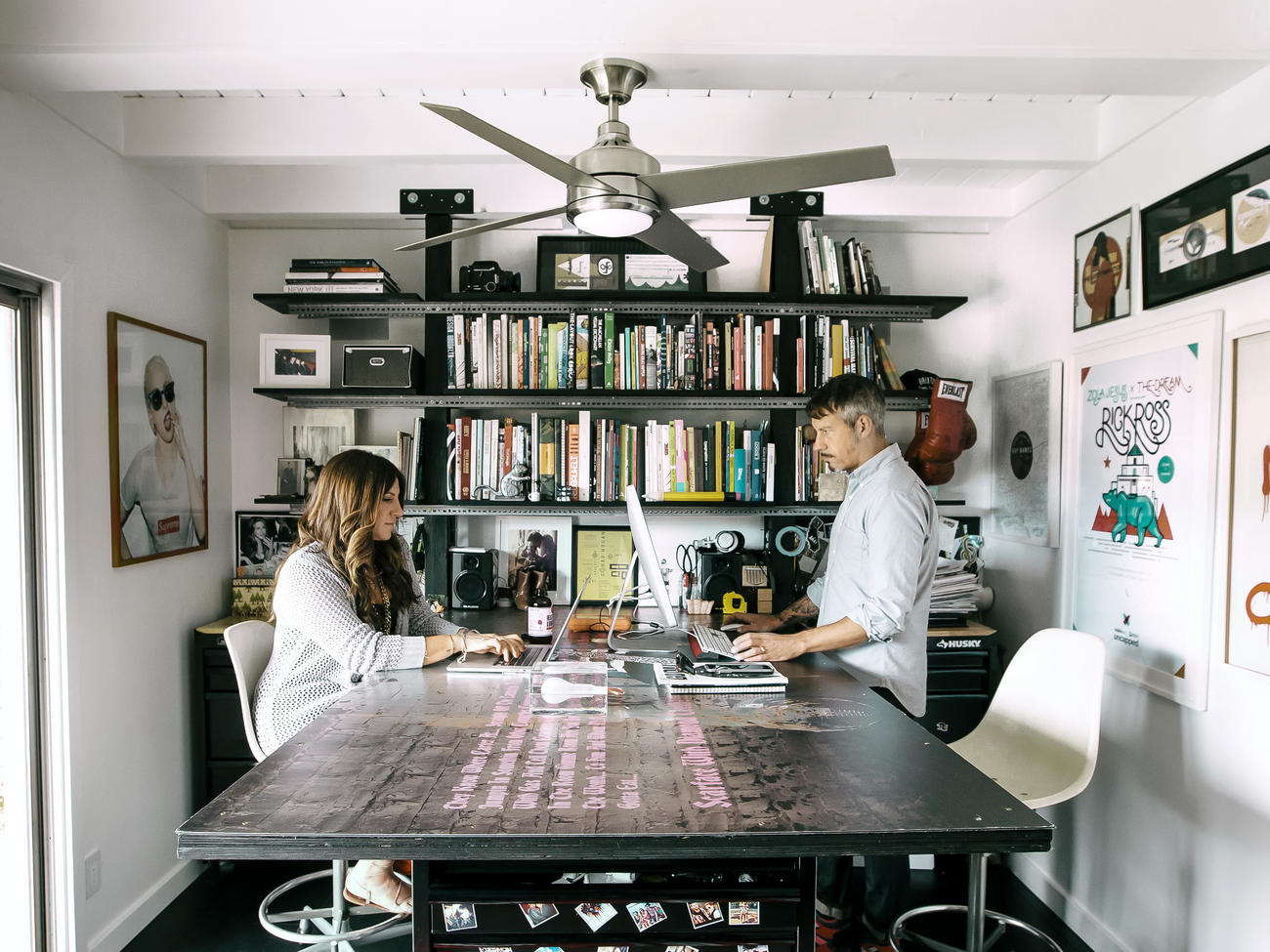This vibrant image, possibly an illustration or digitally enhanced photograph, showcases a modern studio room bursting with color and detail. At the centerpiece is a unique, contemporary table with illegible pink text splashed across its surface. To the left, a woman is seated, busily typing on a laptop, while to the right, a man stands, engaging with a desktop computer and keyboard. The seating in the room consists of minimalist, white, low-set plastic chairs without armrests.

In the background, sleek metal bookshelves line the walls, filled with various items that add character to the space. The walls are adorned with framed pictures and a noticeable "Rick Ross" poster to the right. Adding to the intriguing decor, a pair of boxing gloves dangles behind the man's head. The room's white walls and ceiling, complemented by a silver ceiling fan, enhance the bright, immaculate lighting that illuminates the figures clearly, emphasizing the room's creative and dynamic ambiance.